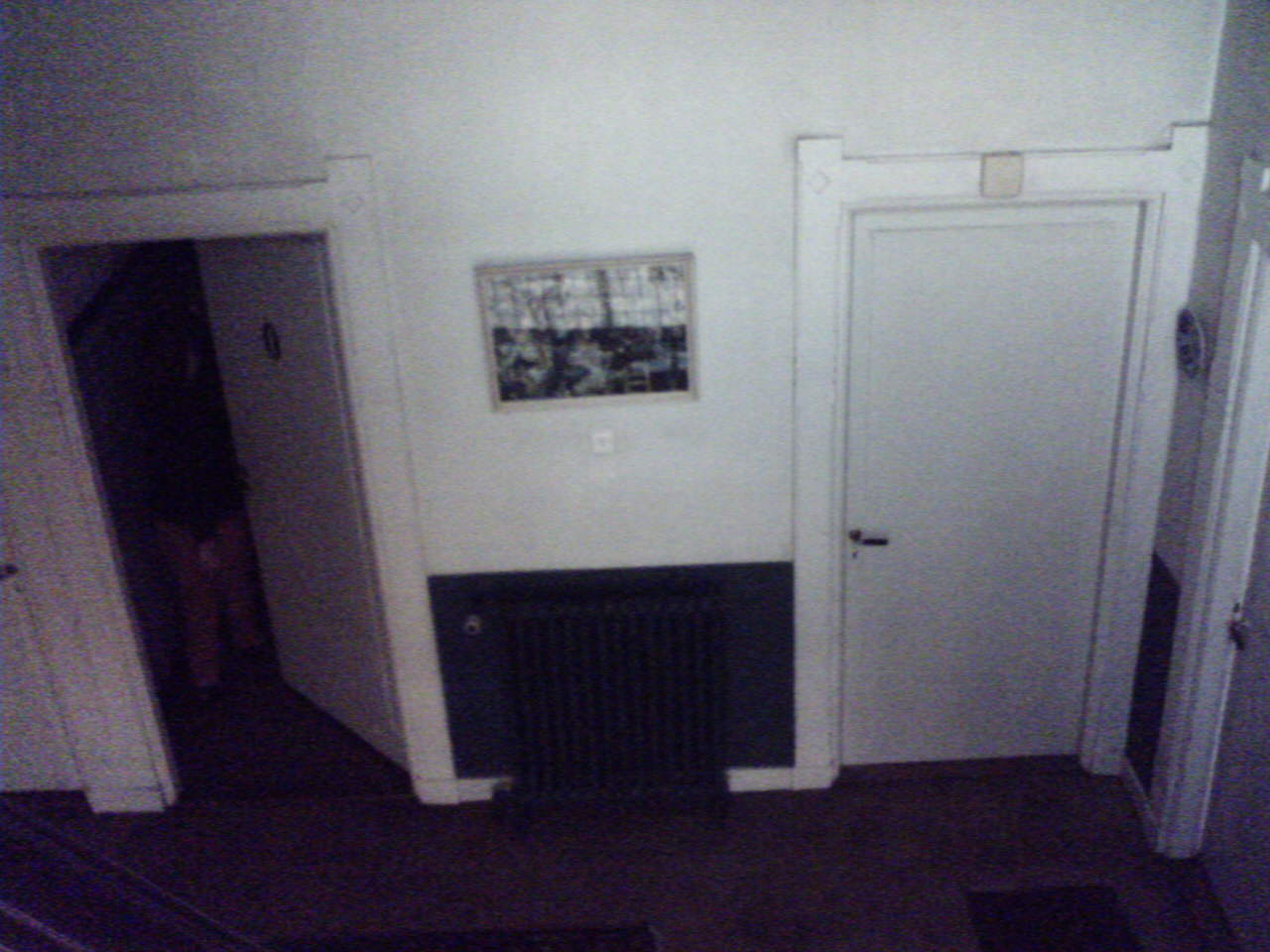This image captures a view from a stairway, looking down at the floor below. The scene features two white doors with wide white frames on either side of a horizontal framed print or photograph mounted on the wall between them. The right door is closed, while the left door is slightly open, angled at approximately 60 degrees. Beneath the photograph, nestled against the wall, sits an old-fashioned steam radiator. Wainscoting adds a touch of classic detailing to the wall around the artwork and radiator. The floor in the scene is a rich dark brown, complementing the lighter tones of the doors and the wainscoting.